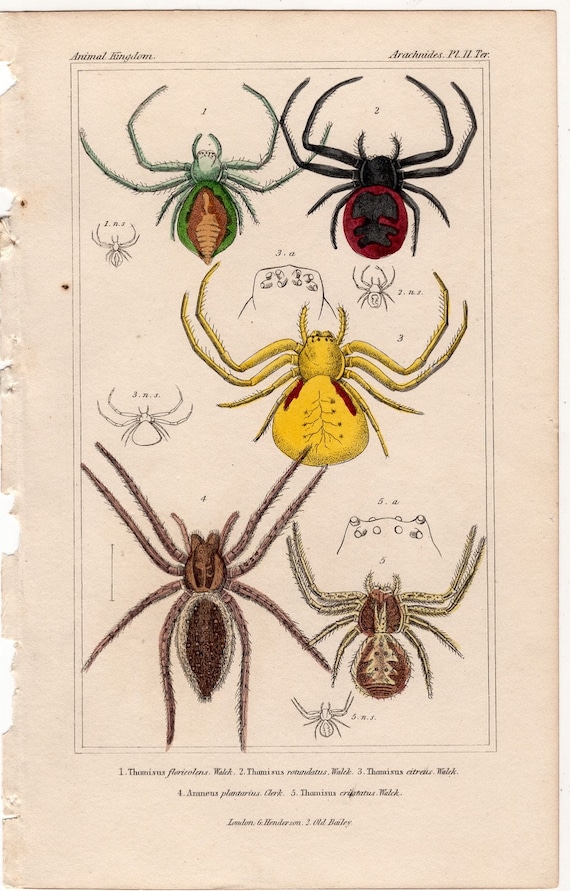This image depicts a detailed diagram from a book about arachnids, specifically focusing on various spider species. The book page has a beige background. At the top of the page, it reads "Animal Kingdom," with "Arachnids Part 2 TER" directly to the right. The central focus is a thin black rectangular box showcasing five detailed spider illustrations. At the top left within the rectangle, there is a green spider with an orange and green speckled body, lighter green hairy legs, and pincers. Opposite it, on the top right, is a black spider featuring a dark blood-red abdomen with a teddy bear shape in the center and black hairy legs and pincers. 

Below these, centered slightly to the right, is a predominantly yellow spider with red stripes near its head and black vein-like patterns on its abdomen. Towards the bottom left of the rectangle is a larger spider resembling a wolf spider or brown recluse. Its abdomen transitions from dark brown in the center to a lighter brown and nearly tan at the edges. The spider's head, legs, and pincers are light brown. On the bottom right, there's a smaller spider with a light brown abdomen, a tannish white Christmas tree shape in the center, and darker brown edges. This spider also has similarly colored legs and pincers that are hairy.

Each spider is illustrated from a top-down perspective, and the bottom of the page includes a small-font key indicating the species names, though the text is too tiny to read clearly. The image provides a mix of color and grayscale illustrations, effectively capturing the diversity among spider species, from body colors and patterns to variations in leg lengths.